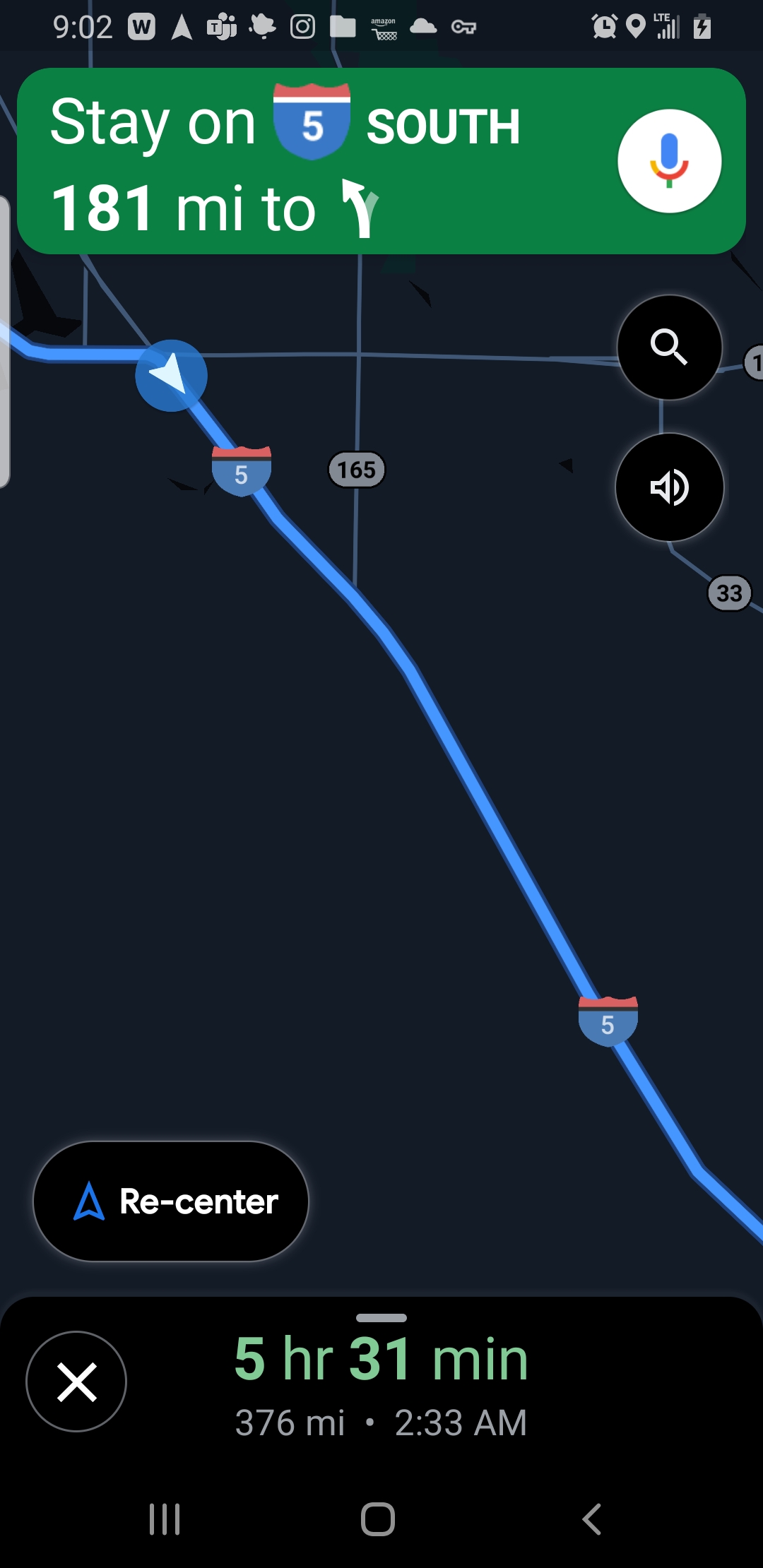This image appears to be a screenshot of a GPS navigation screen from a smartphone. The top of the screen displays multiple icons: a Weverse app icon, a GPS icon, a friend group icon, a weather icon, an Instagram icon, a folder icon, and a key icon. The time is shown as 9:02, although it does not specify a.m. or p.m. The battery level is approximately 90%, and the device has four bars of signal strength. An alarm has been set, and the location service is active.

The main navigation display advises to "Stay on Interstate 5 South, 181 miles to a left-hand exit," presented on a green background. Adjacent to this text, there is a microphone icon in blue, gold, and black; the microphone itself is blue, the holder is gold, and the stand is black.

The map is depicted in dark blue, featuring Interstate 5 and its intersection with Route 165. The map does not specify the exact road for the left turn 181 miles ahead, suggesting continued travel on I-5 South. At the bottom of the screen, a recenter icon is visible. The navigation details indicate a travel distance of 376 miles, an estimated duration of 5 hours and 31 minutes, and an estimated time of arrival at 2:33 a.m.